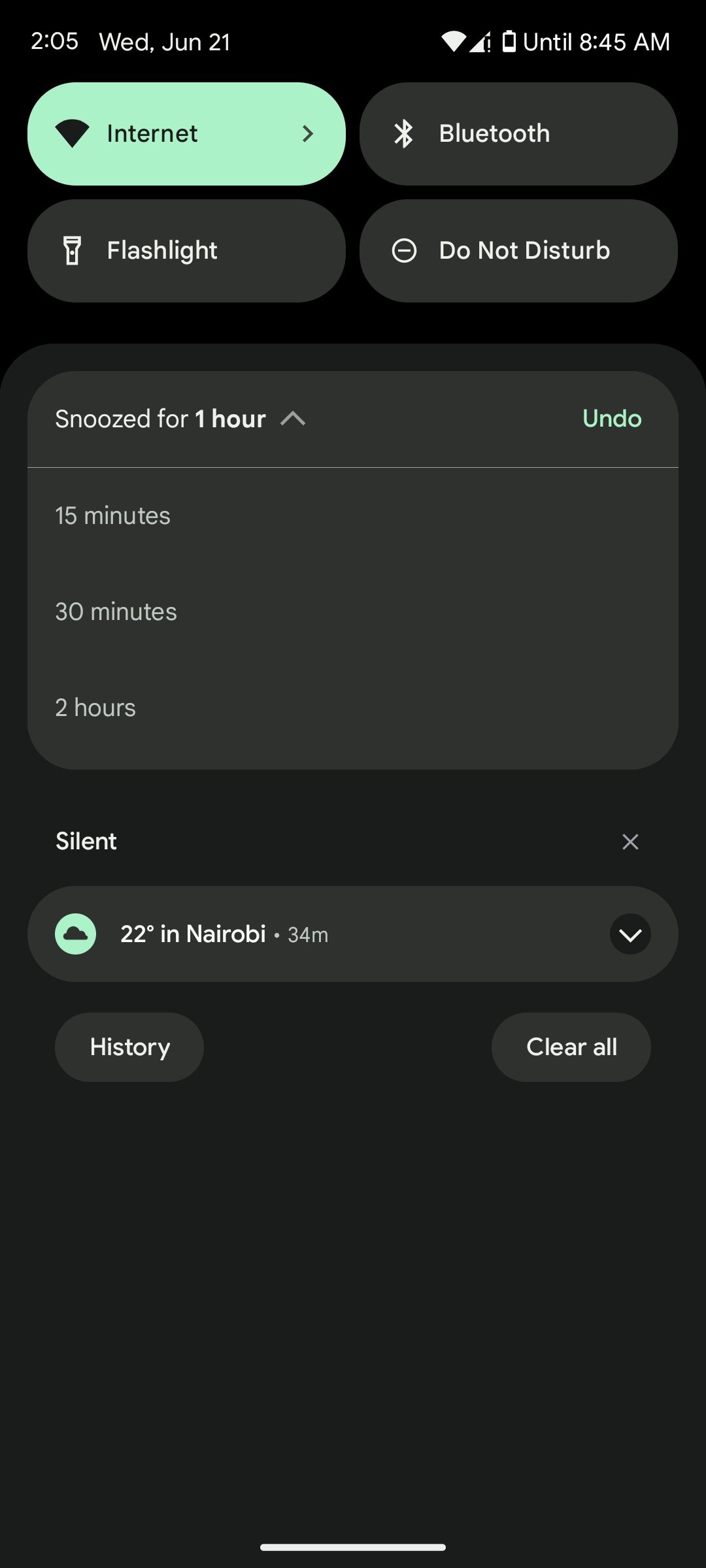This is a detailed screenshot from a mobile phone display. The background is predominantly black. At the top-left corner, it shows the time "2:05" in white alongside the day and date: "Wednesday, June 21st." Moving right, it displays the battery icon, nearly empty with just a sliver of white across the bottom, indicating low battery. Beside it, there are two icons representing wireless connectivity: one shows the internet signal at half strength, and the other shows full WiFi connectivity.

Below the time and date, on the left side, there is a small teal-green tab featuring a black WiFi icon, labeled “Internet” with a right-pointing greater-than symbol next to it. Adjacent to this is a black tab with a Bluetooth icon labeled “Bluetooth.” Further down on the left, there is a grey tab with a flashlight icon labeled “Flashlight.” Another grey tab below features a circle with a line through it, labeled “Do Not Disturb.”

A large grey square occupies the middle section of the screenshot. At the top-left of this square, it reads "Snoozed for one hour" with an upward-pointing greater-than sign. On the top-right, it displays an "Undo" option. Below this text, a line separates the top section from the bottom, where it reads "15 minutes" followed by "30 hours" indicating settings for the alarm.

Returning to the black background beneath the grey square, the left side shows "Silent," and the right features an "X." At the bottom, there is a grey search bar spanning from left to right. Inside the search bar, on the left, a green circle with a black cloud icon is displayed next to text indicating "22°C in Nairobi, 34M." Below the search bar, on the left, a grey tab labeled "History" in white text can be seen, with a corresponding grey tab on the right that reads "Clear All."